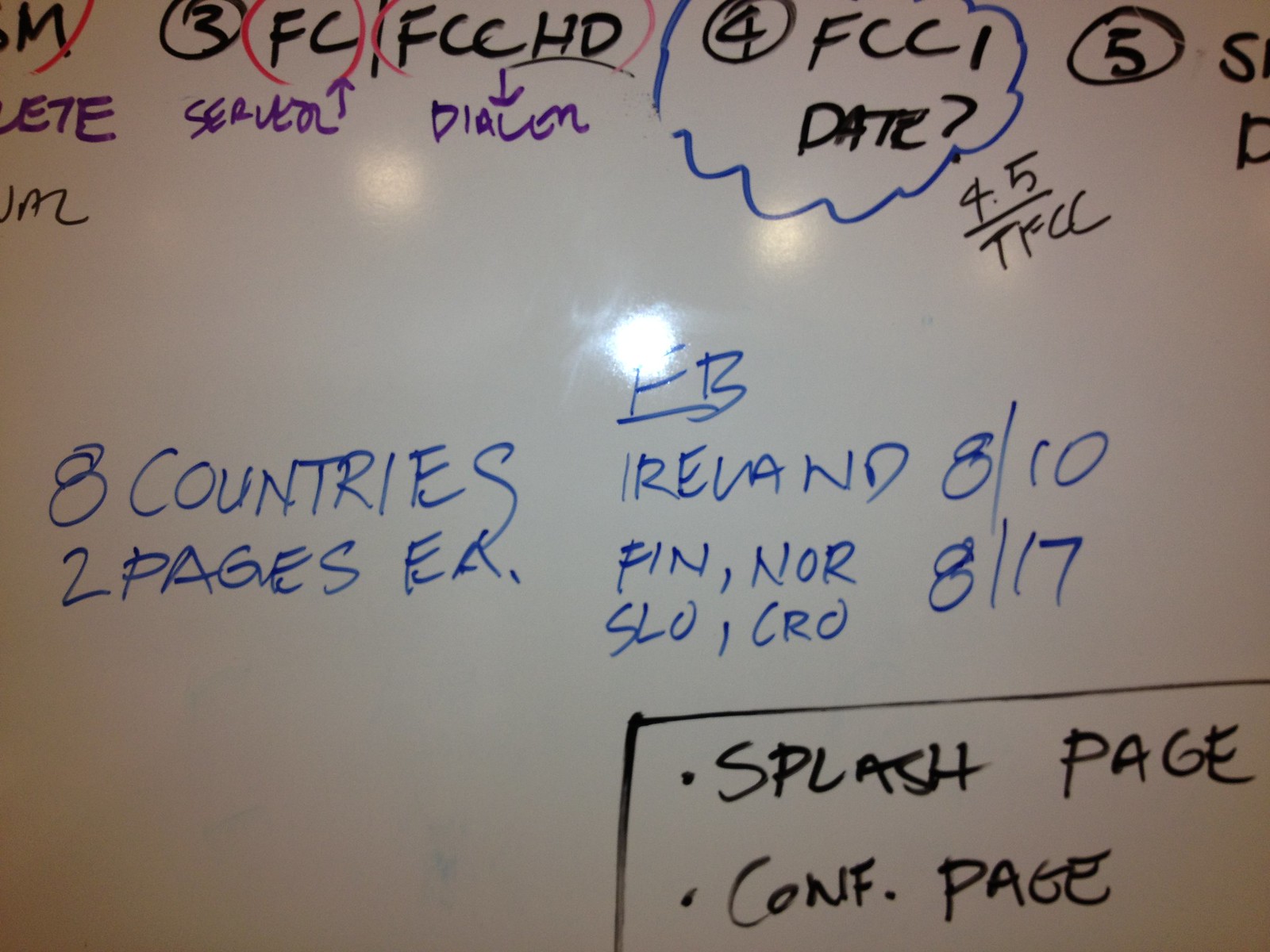The photograph captures a whiteboard covered with various notes and diagrams, seemingly from a college or office setting. At the top, in black letters, are cryptic alphanumeric strings such as "3FCFCCHDFCCID?4.5TFCC5" and "FCC HD," some of which are encircled in red. A date is also present with a question mark. In purple lettering, "ETE server" points upward with an arrow, and "DILM" points downward with another arrow. Centrally, the board lists "8 countries, 2 pages EA," with specific countries like Ireland ("8 out of 10"), Finland, Norway, Slovakia, and Croatia ("8 out of 17"). There is also mention of "8 bar 11" and the title "EB." On the bottom right corner, written in black, are items "splash page" and "conference page," noted as a list. The photo also shows a reflection of room lights, including one prominent flash at the center of the board and three faint ones at the top. Numerous markers in black, blue, red, and purple colors are used throughout, and the image seems to capture only a portion of the whiteboard.